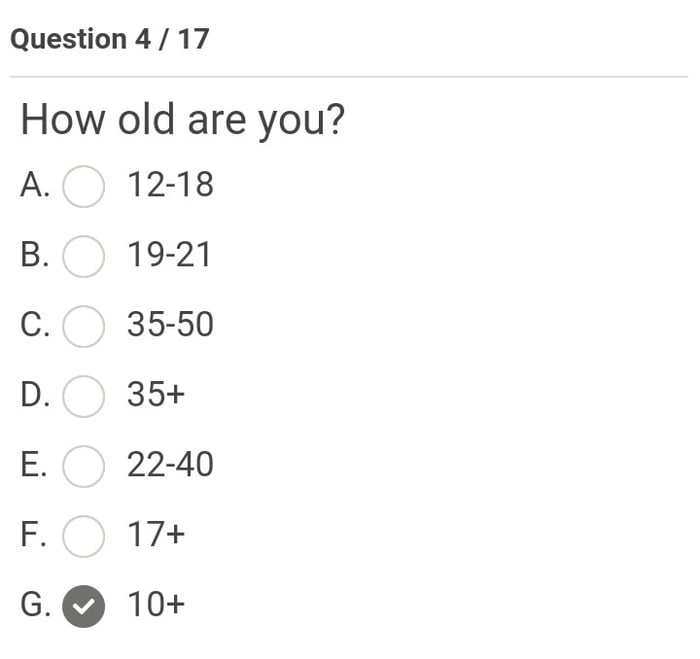The image depicts a form with a series of questions, specifically highlighting Question 4 out of 17. The question asks, "How old are you?" and provides a set of age ranges each accompanied by a selection bubble. The options listed are as follows:

- Option A: "12 through 18"
- Option B: "19 through 21"
- Option C: "35 through 50"
- Option D: "35 plus" (Note: This option is ambiguous due to the overlap with Option C)
- Option E: "22 through 40"
- Option F: "17 plus"
- Option G: "10 and up" (This option is checked)

This confusing overlap in age ranges appears to be designed to test the attention and self-perception of the respondent. For example, a 36-year-old could potentially select any one of the following options: "35 through 50," "35 plus," "22 through 40," "17 plus," or "10 and up." The form presents a nuanced challenge in determining the most appropriate selection, given multiple categories that apply to the same age groups.